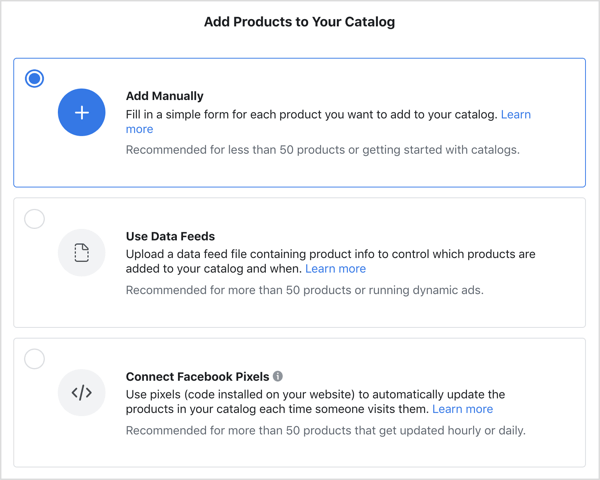This image is a screen capture of a web page, likely related to e-commerce or digital catalog management, featuring a predominantly white background with black text. The layout is divided into three horizontal rectangular sections, one stacked above the other.

At the top of the page, in the first section, is a title in bold that reads "Add products to your catalog." This section is labeled "Add Manually" and includes a blue dot in the upper left corner along with a blue circle containing a plus sign. The accompanying text states: "Fill in a simple form for each product you want to add to your catalog." Following this is a "Learn more" link in blue. This option is recommended for adding less than 50 products or for getting started with catalog management.

The middle section is not selected and is labeled "Use Data Feeds." It features an icon depicting a document within a circle. The instructions indicate that users can upload a data feed file containing product information to manage which products are added to the catalog and when. This section also includes a "Learn more" link. It is recommended for adding more than 50 products or for those running dynamic ads.

The bottom section, also unselected, is titled "Connect Facebook Pixels" and includes an icon that likely represents Facebook Pixels. It explains that users can "use pixels (code installed on your website) to automatically update the products in your catalog each time someone visits them." A "Learn more" link follows this description. This method is recommended for catalogs with more than 50 products that require hourly or daily updates.